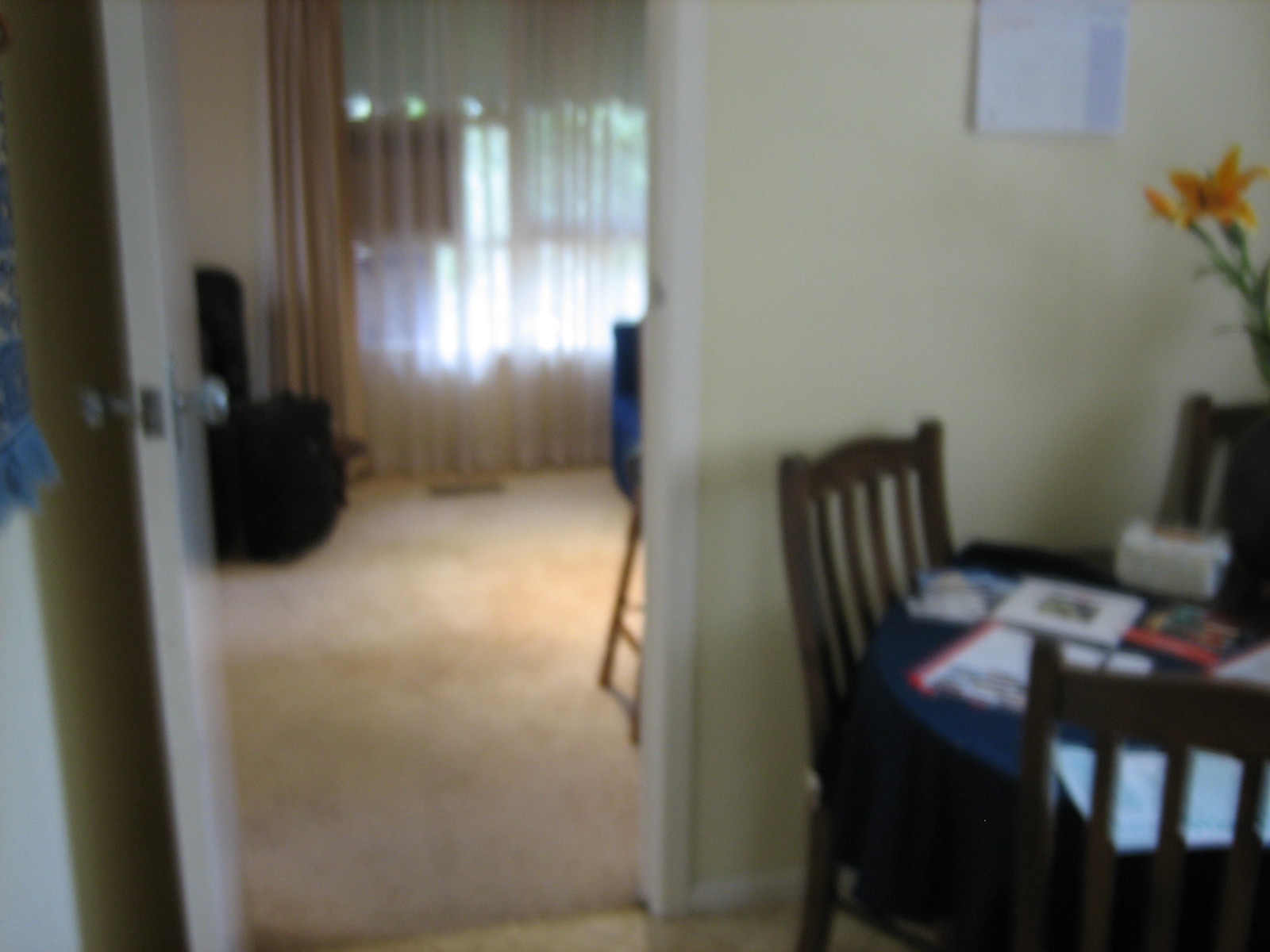The image portrays a cozy interior scene captured from one room, looking through a doorway into an adjoining room. In the foreground, there is a table draped with a blue tablecloth and adorned with white objects that appear slightly blurred. Surrounding the table are wooden chairs, adding a touch of warmth to the setting. A vibrant flower with orange petals is also visible, adding a pop of color to the scene. A picture frame or similar wall decor is mounted on the wall behind the table.

Peering through the doorway into the next room, a light brown carpet is visible, grounding the space. In the corner, a black reclining chair beckons with a promise of comfort. The window in this room is adorned with sheer white curtains, allowing light to filter through softly. Additionally, a partially visible chair with a blue back and wooden legs can be seen, enhancing the room's inviting atmosphere.